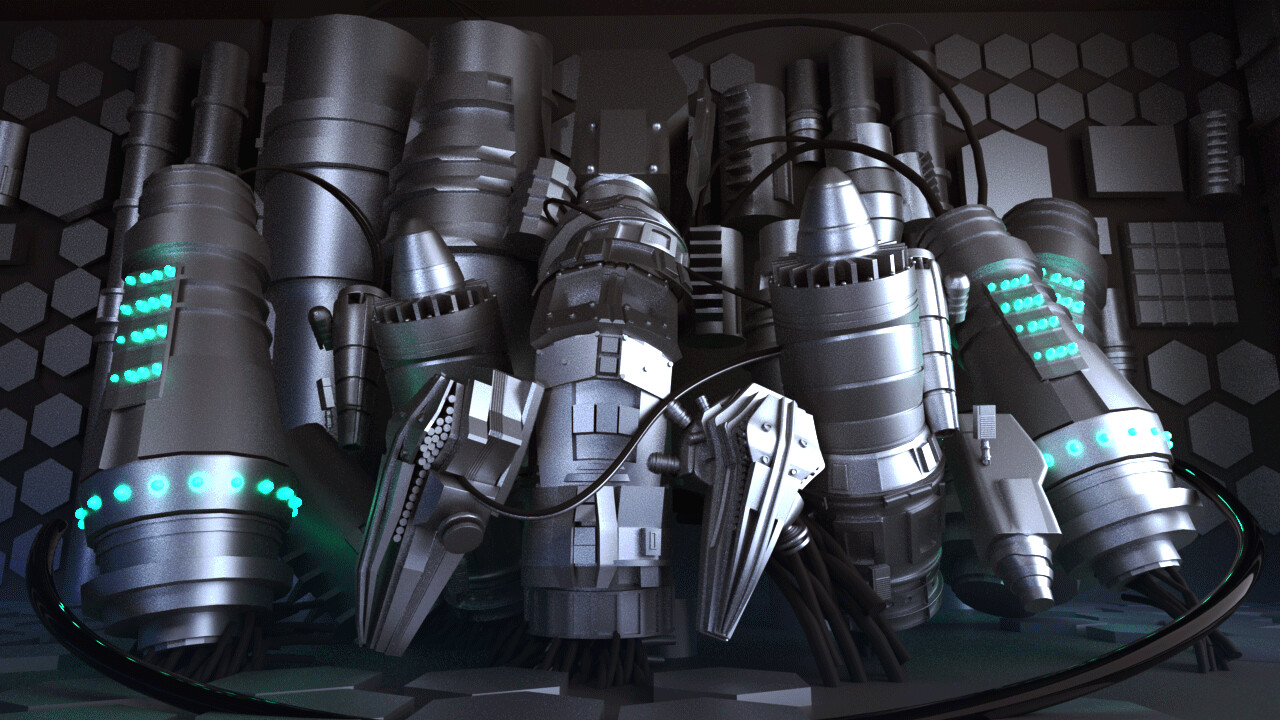This horizontal digital illustration showcases an intricate array of high-tech machinery parts, characterized by their rounded edges and meticulously detailed design. The central focus is on a series of cylindrical or canister-like devices, finished in a sophisticated palette of silver and gray, accentuated with realistic highlights and shading. Each device features glowing green lights, exuding a futuristic ambiance reminiscent of spaceship control panels. These sleek, robotic components are arranged symmetrically on the left and right sections of the composition, each residing within a prominent black circular frame. Surrounding these main elements are additional robotic parts, further enhancing the complexity of the scene. Flanking the image on both sides is a border of interconnected six-sided shapes, forming a honeycomb pattern that adds an extra layer of geometric precision to the overall design.